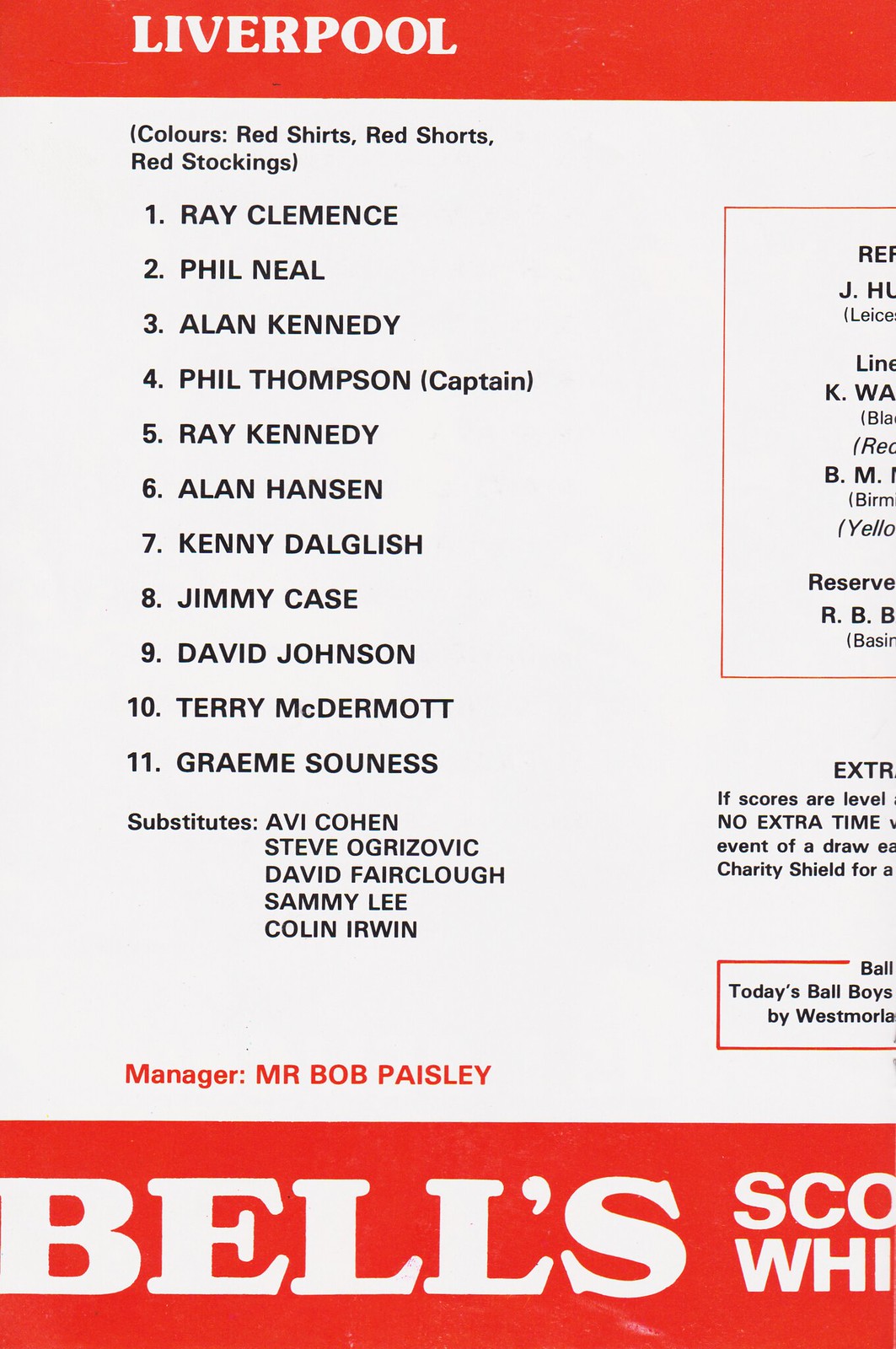This is a scan of what seems to be a page from a program or magazine. Dominating the top section is a red banner with white, capitalized text reading "Liverpool." Below this, in the larger, predominantly white middle portion, black text in parentheses lists the team's colors: "Red shirts, red shorts, red stockings."

The page continues with a numerical list of players: 
1. Ray Clemence 
2. Phil Neal 
3. Alan Kennedy 
4. Phil Thompson, captain 
5. Ray Kennedy 
6. Alan Hansen 
7. Kenny Dalglish 
8. Jimmy Case 
9. David Johnson 
10. Terry McDermott 
11. Graeme Souness

There is a mention of substitutes, listing A.B. Cohen, Steve Ogrizovic, Steve Fairclough, Sammy Lee, and Colin Irwin. Some text on the right side of the page is partially cut off. 

At the bottom of the page, in red letters against a white background, is the manager’s name: "Mr. Bob Paisley." Concluding the page, another red section with white text includes the word "Bells," which seems to be part of a longer, incomplete phrase.